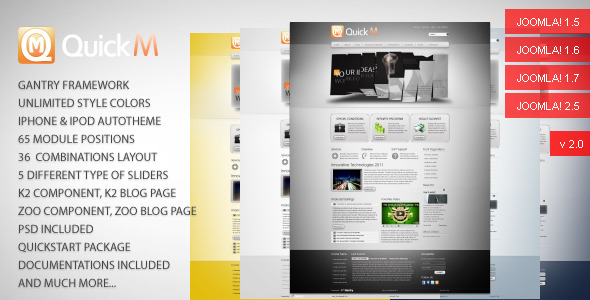This vibrant, computer-generated advertisement showcases the extensive features of "Quick M." The brand logo is eye-catching: an orange square framing a stylized white "Q" with an "M" embedded in its center. Below the logo, a detailed list of features is displayed, including a gantry framework, unlimited color styles, auto themes for iPhone and iPod, 65 module positions, 36 layout combinations, five different sliders, K2 component and blog page, Zoo component and blog page, PSD files, a quick start package, comprehensive documentation, and more.

To visually represent these offerings, the ad features five distinct screenshots displaying various framework styles. These frameworks differ in color: gray, white, yellow, light gray, and blue. Each represents the diverse display features provided by Quick M, despite their similar layouts. Along the right side of the ad, compatibility with multiple Joomla versions is highlighted, listing Joomla 1.5, 1.6, 1.7, 2.5, and 2.0. The ad effectively communicates the robustness and versatility of Quick M, catering to users seeking a comprehensive and customizable web development solution.